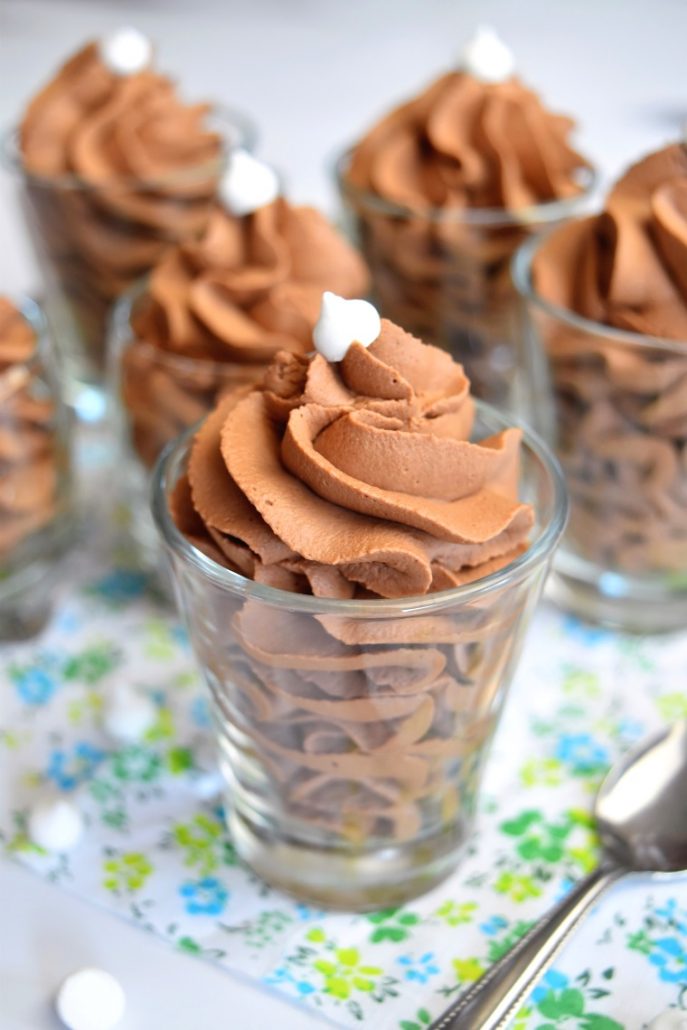The photo illustrates six small, clear glasses arranged on a tablecloth adorned with blue and yellow floral patterns and green leaves. Each glass is filled with a swirled brown dessert, likely mousse or ice cream, topped with a single white chocolate chip. Scattered around the glasses are additional white chocolate chips, resembling small decorations. A silver spoon rests in the bottom right corner of the image. The background appears slightly blurred, drawing attention to the detailed textures and colors of the desserts and tablecloth in the foreground.